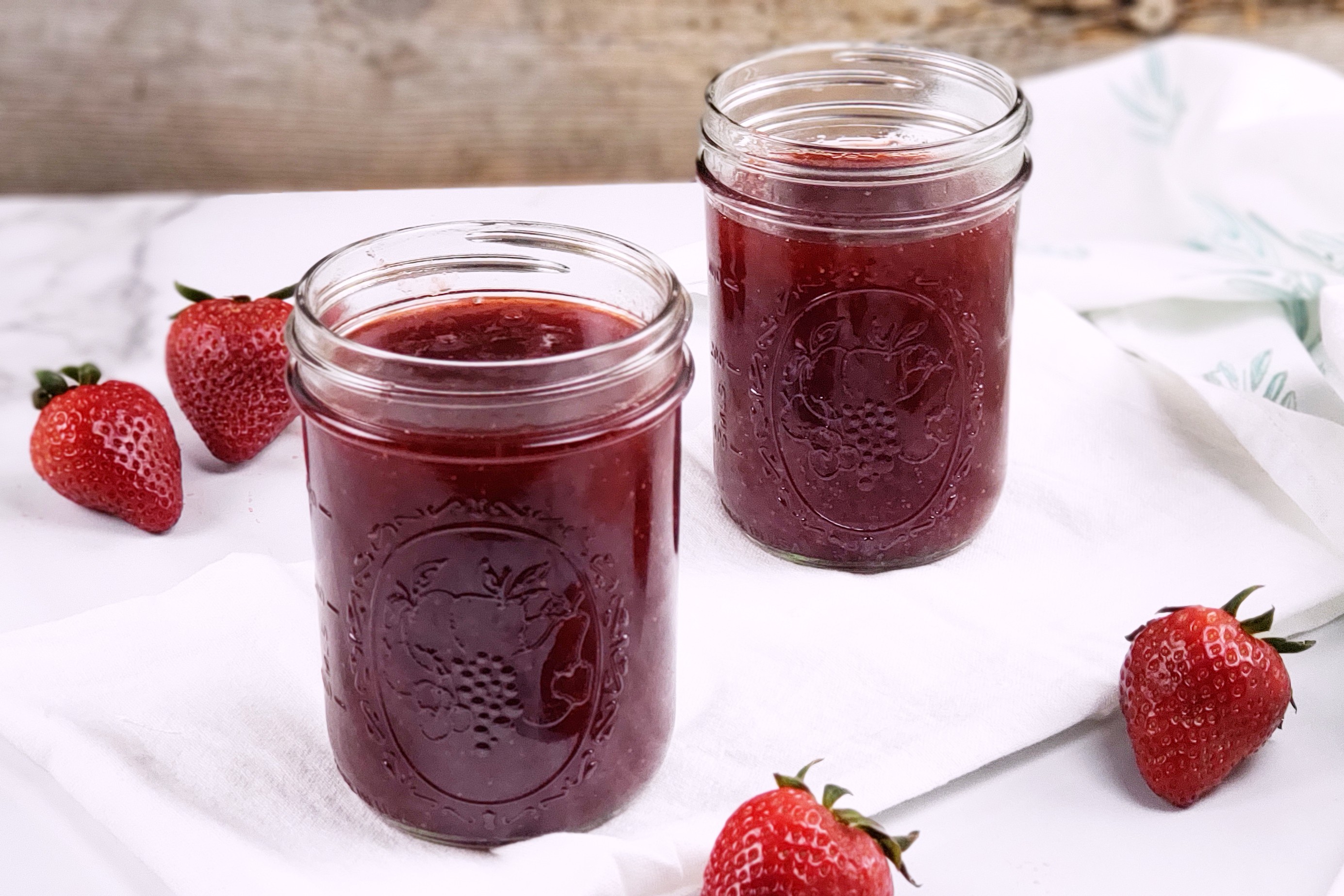This realistic, horizontally oriented photograph features two elaborately designed glass mason jars filled with deep red strawberry jam, positioned without their lids. Each jar is embellished with intricate engravings of fruits and leaves. Surrounding the jars artistically are four ripe strawberries, two on the left and two on the right, their vibrant red hue and green leaves providing a striking contrast to the jam. The setup is arranged on a white cloth, possibly placed on a wooden surface that serves as a subtle background. This visually appealing arrangement suggests a display for promoting homemade strawberry jam, perhaps ideal for a farmers market or a social media post, with its clean, inviting presentation and wholesome aesthetic designed to attract attention and appreciation.